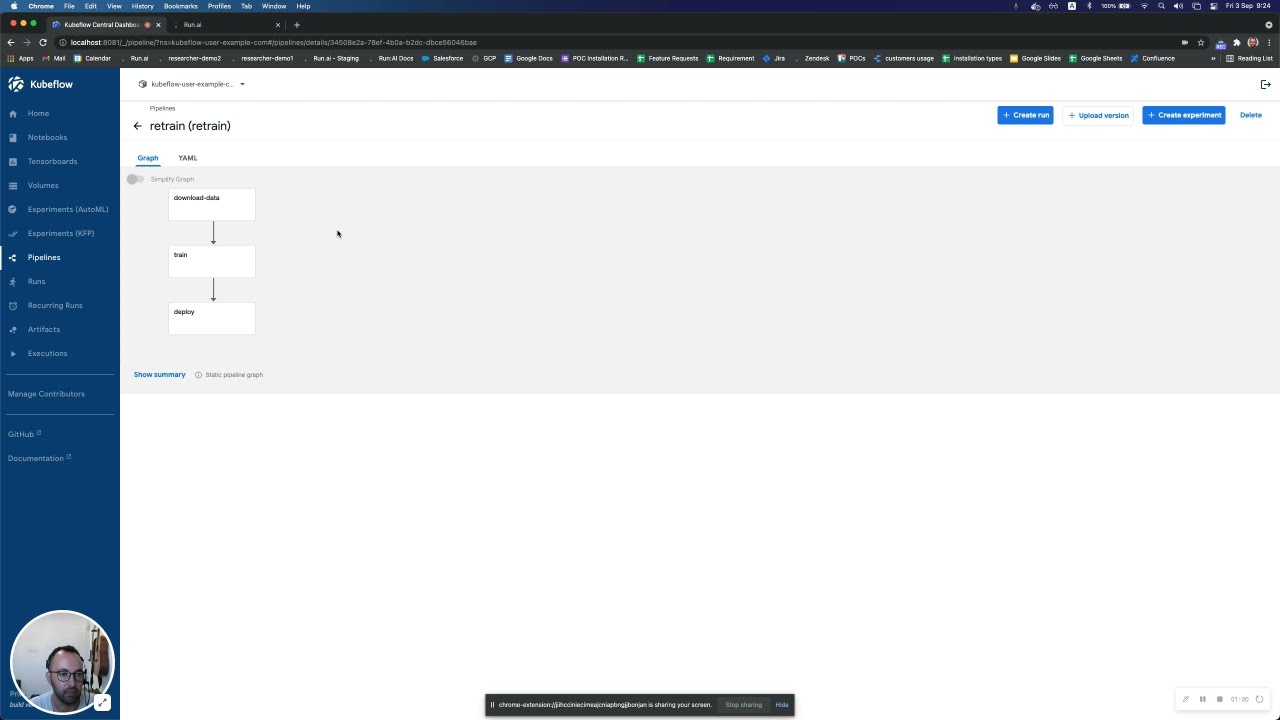In the image, we are viewing a somewhat unclear website with parts of the content in another language. Dominating the left side of the screen is a prominent blue panel featuring a long rectangle that seemingly displays "Coots Flow" in white letters at its top left corner. Adjacent to this panel is the primary section of the website, which is relatively sparse in information. The word "Retrain" appears in black letters, followed by text that might spell out "O-R-E-T-R-A-I-N" or a translation of "Retrain" in another language. 

Three blue rectangles are present, with arrows pointing downwards between them. Returning to the blue bar on the left, there is an image at the bottom showing a man wearing glasses and a beard, suggesting this might be a communication-focused website with the individual actively engaged. His image is depicted with clarity. Additionally, there are small, indistinct options at the very top of the page. In the right-hand area but not at the very top, blue and white rectangles appear in an alternating pattern.